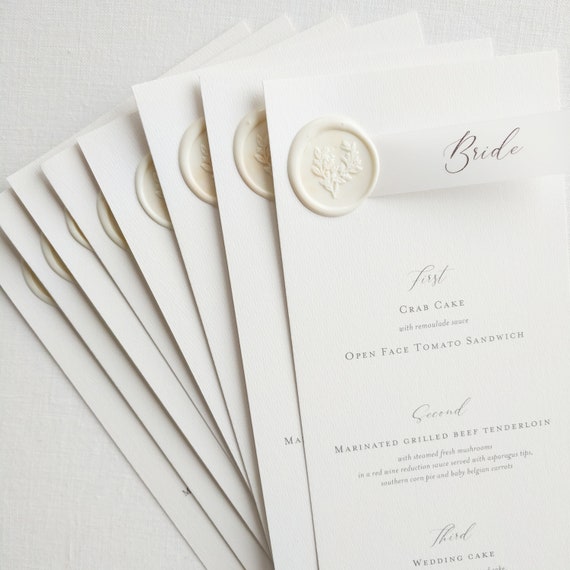The image depicts a set of eight elegantly designed wedding menu cards laid out against a grayish-white background. Each card, adorned with a cream-colored wax seal bearing a leaf design, showcases refined calligraphy at the top spelling out "Bride." The menu is divided into three courses. The first course features a crab cake with remoulade sauce alongside an open-faced tomato sandwich. The second course offers a marinated grilled beef tenderloin with steamed fresh mushrooms in a red wine reduction sauce, accompanied by asparagus tips, southern corn pie, and baby Belgian carrots. The final course consists of a wedding cake. These cards are stacked in such a way that we can clearly read the detailed menu on the top card, with hints of the same content visible on the others.